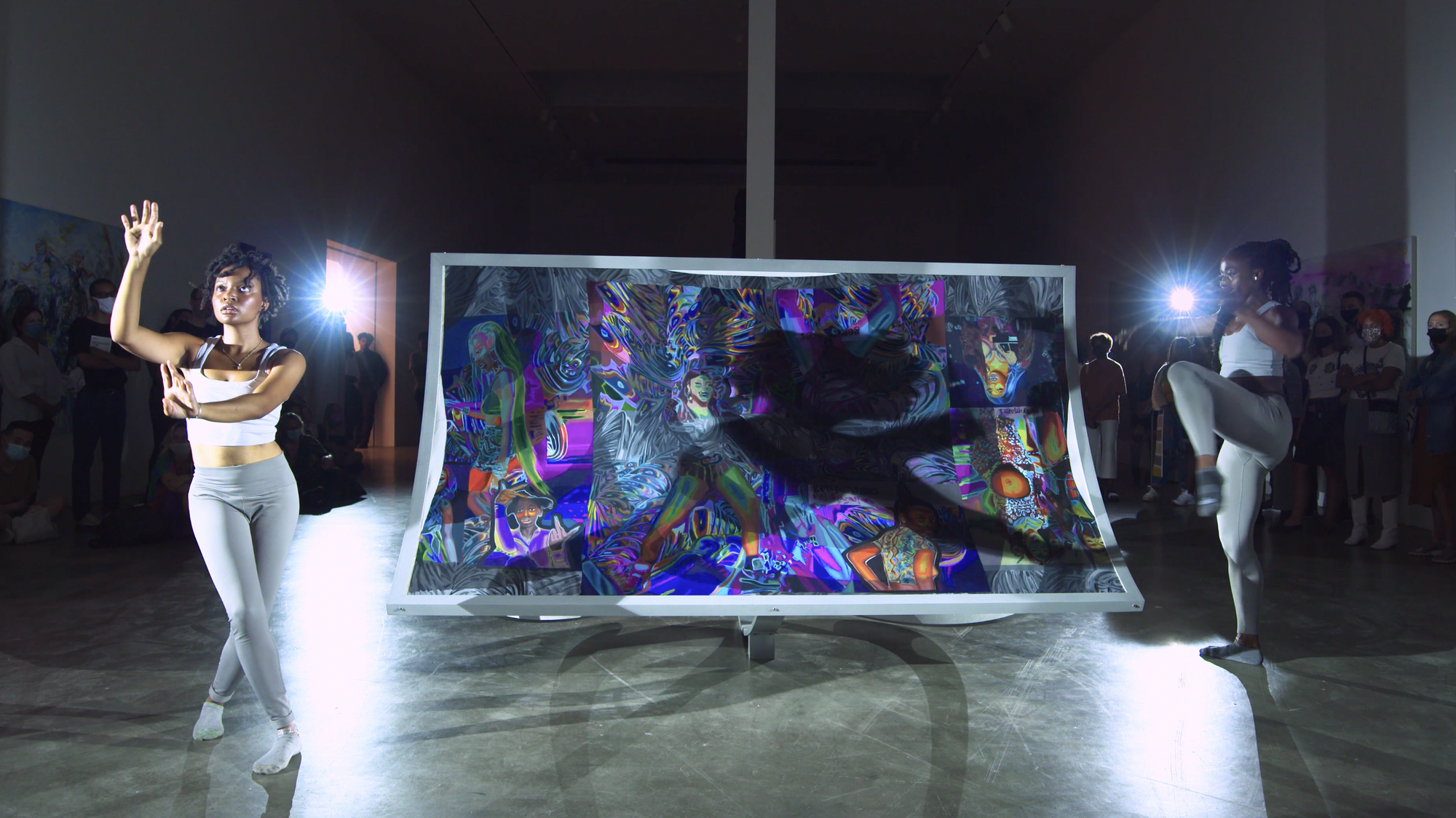In the center of this vibrant color photograph, two African-American women are performing a dance in an art gallery. They are both dressed in white tank tops, gray tight-fitting leggings, and white socks. One woman, positioned on the left, has short hair and looks upwards with her left hand raised and her right hand stretched out in front of her, capturing an ethereal moment. The other woman, on the right, has long braided hair pulled back and is mid-movement, with her left knee bent up toward her chest, as if preparing to kick something.

Behind them, a large canvas adorned with an abstract, psychedelic painting in bright hues of purple, blue, hot pink, red, and orange captures the eye. The artwork includes various figures; among them, a person in the bottom left corner pointing with a middle finger, a woman with dreads on the upper left, another woman dancing in the center, and a woman facing the opposite direction in the bottom right corner.

The performance is illuminated by bright spotlights, which cast dramatic shadows across the painting and add depth to the image. The gallery is dimly lit, focusing attention on the dancers and the vibrant painting, while the audience remains in the shadows. Observers, who seem to be wearing masks indicative of the COVID-19 period, watch the performance intently from the darkness, their faces obscured, adding a sense of mystery and intensity to the scene.